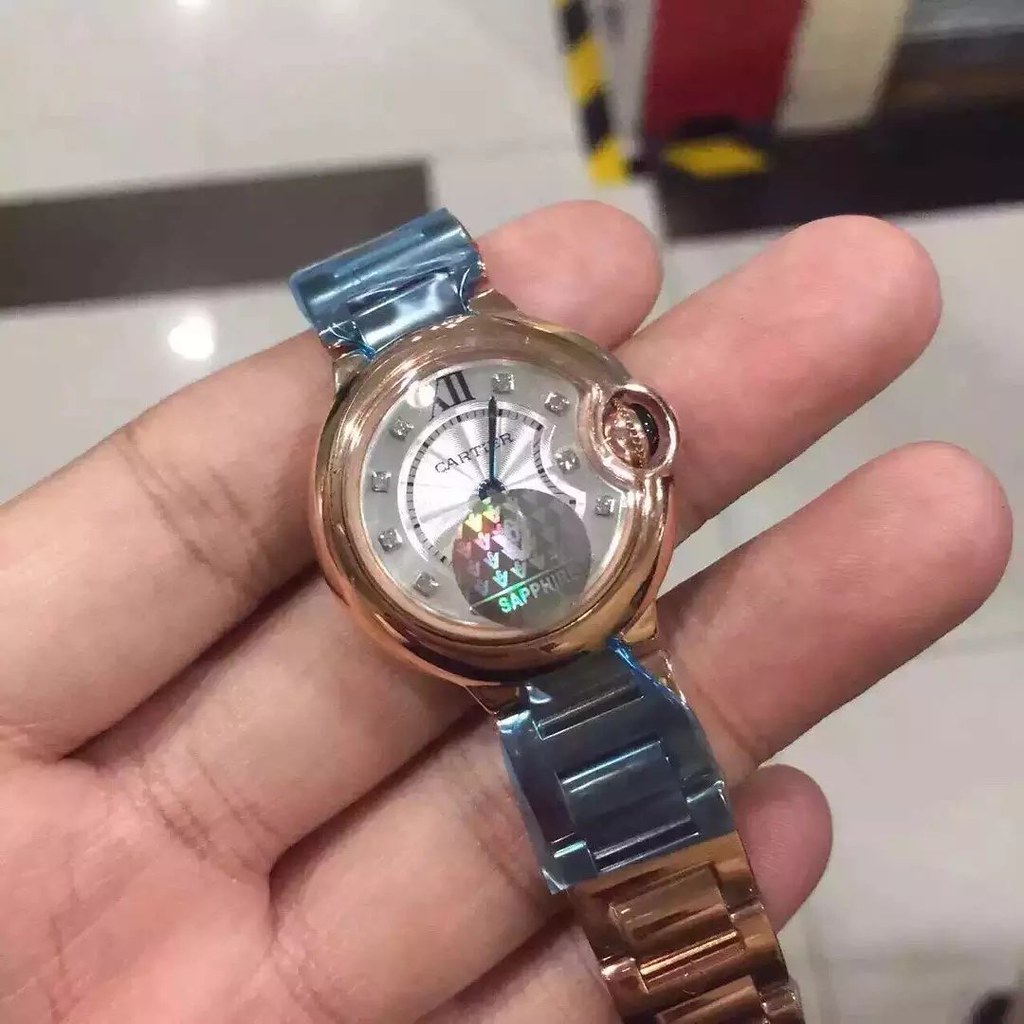In this detailed close-up photograph, a white male is seen holding a luxurious gold Cartier watch in his open hand, resting on his fingertips, which are visibly spread out. The watch, characterized by its all-brass construction, features a glass dome over the silver timepiece adorned with Roman numerals and small diamond chips. The face of the watch displays a single hand, almost pointing at one, and prominently showcases a gold dial. Notably, a holographic circular sticker with the word 'Sapphire' can be seen affixed over the numbers six and seven, adding a disco-like vibe. The watch band consists of galvanized brass at the top, transitioning into a solid brass band. Some remnants of its original blue protective shrink wrap are still visible, emphasizing its newness. The setting includes a white background with a faint glimpse of a tile floor, and what appears to be an elevator entrance is partially visible in the upper right-hand corner.